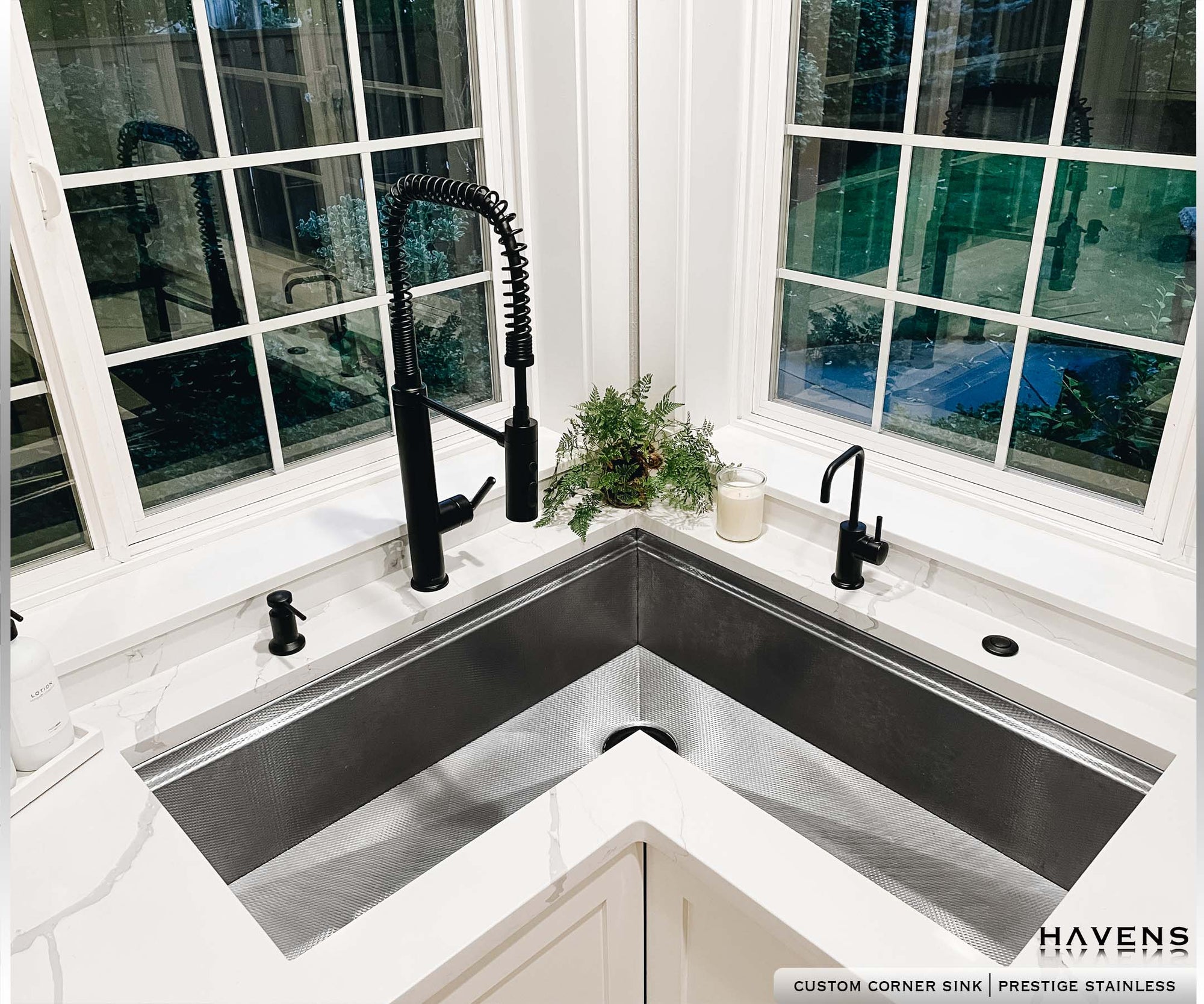The image captures a corner of a modern kitchen featuring an L-shaped stainless steel sink. The sink has a tall faucet on the left side and a smaller faucet, likely a soap dispenser, on the right side. The countertop is white with gray veining, resembling marble. Above the sink, there are two white-framed windows that reflect the kitchen interior. In the corner, small green plants and a white candle adorn the windowsill. The area underneath the sink showcases a mix of black and white cabinets. Notably, a text in the bottom corner indicates "Haven's Custom Corner Sink Prestige Stainless" in black font.